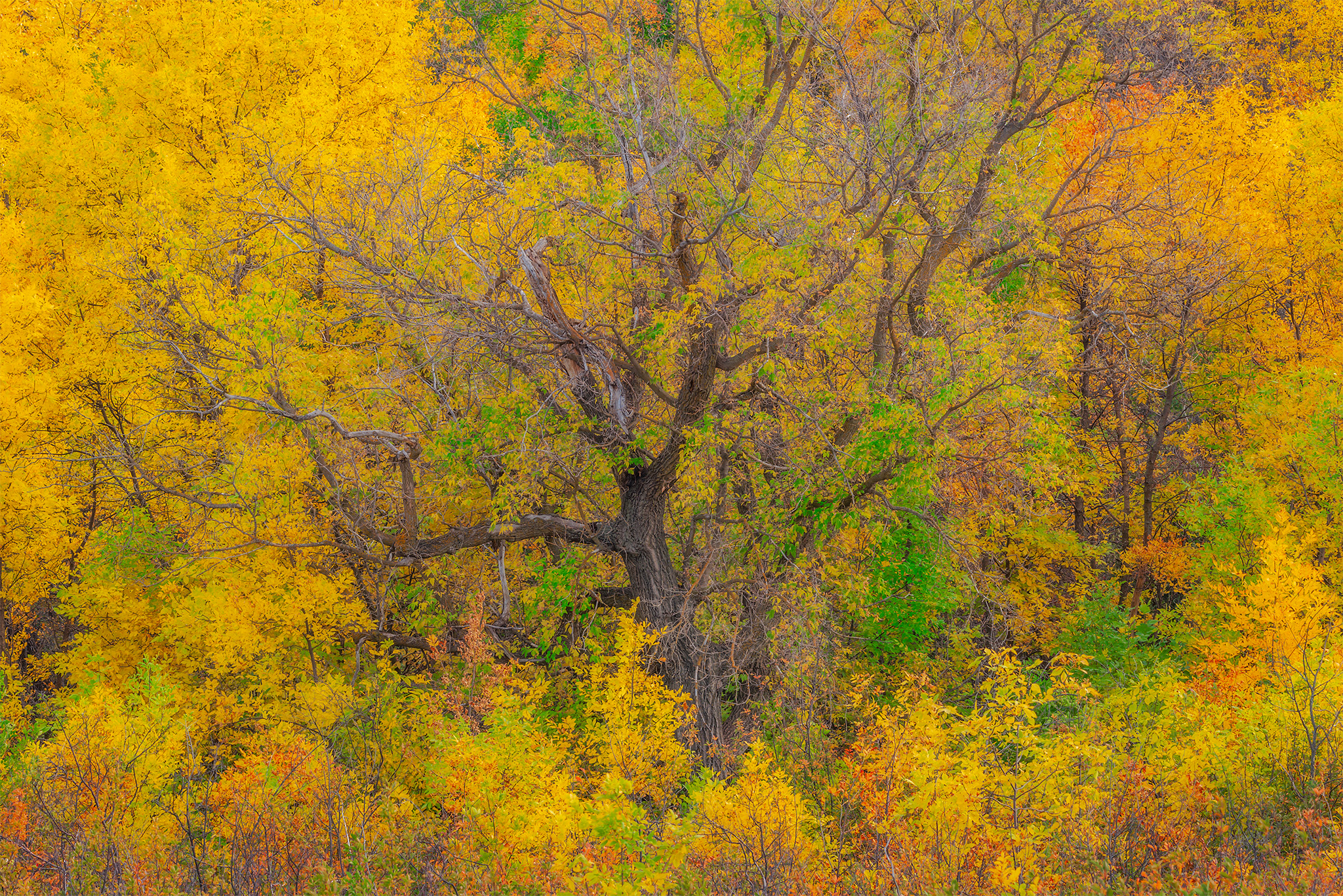This detailed photograph showcases a dense forest during the peak of autumn, where the majority of the trees flaunt vivid yellow foliage, with interspersed splashes of green and orange. A prominent, large tree with a notably thick trunk stands out in the center, dwarfing the numerous smaller trees surrounding it. The setting appears to have been slightly color-corrected or enhanced, giving the leaves an even more vibrant hue. The close-up perspective reveals an intricate network of limbs and branches, with bark in dark brown hues, contributing to the overall autumnal tapestry. Despite the vividness of the foliage, the scene is naturalistic, emphasizing the richness and intensity of fall colors during the daytime. The forest canopy fills the entire frame, creating an immersive experience of the seasonal transformation.